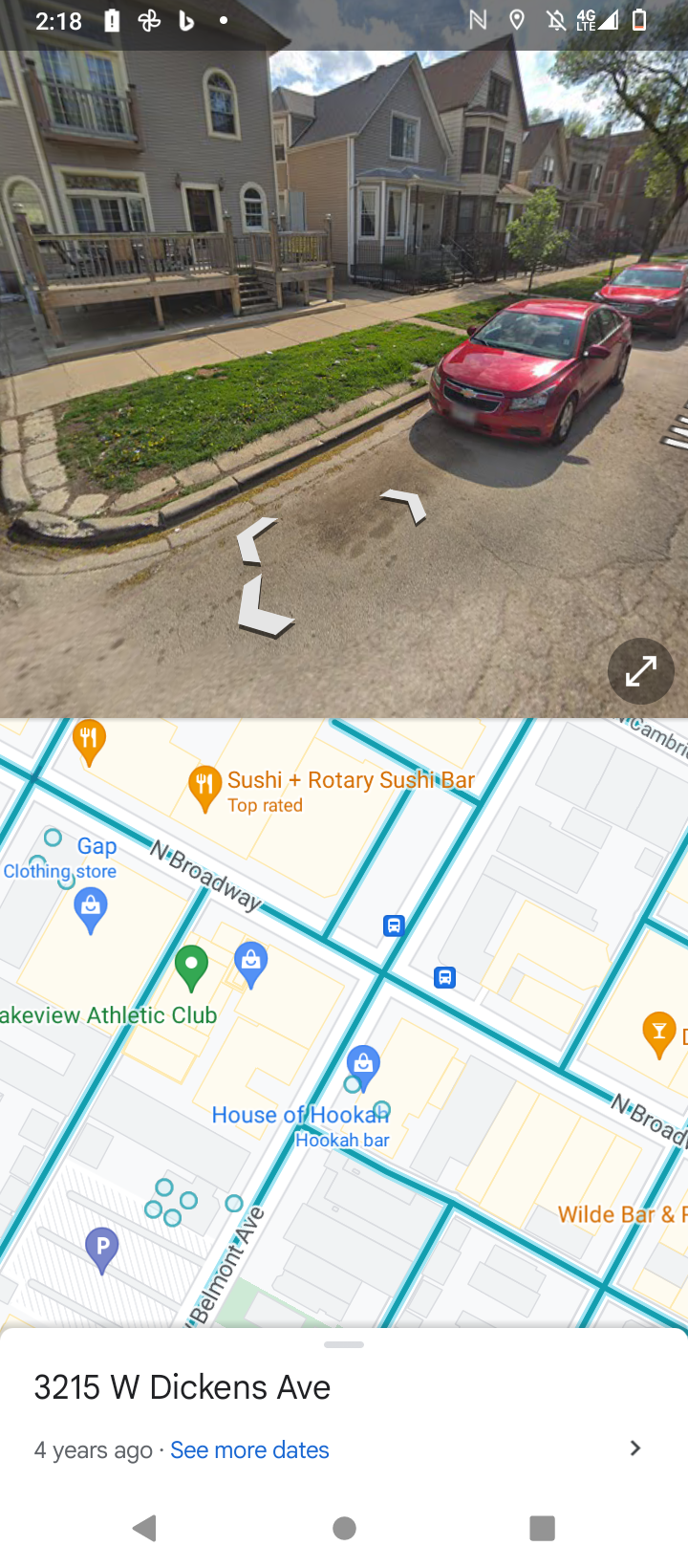This image depicts the results of a Google search on an iPhone, captured around four years ago. The screen is split into two sections. The top half showcases a photo of a two-story house or condominium located at 3215 West Dickens Avenue. In front of the house, there is a small wooden deck and a narrow sidewalk, bordered by a modest grass area. Two red cars are parked on the street nearby. The house is part of a series of similar-looking two-story homes, with adjacent houses visible on either side. The bottom half of the screen features a map highlighting various businesses. North Broadway Street is prominently displayed, along with several other intersecting streets marked with pinpoint icons denoting different establishments.